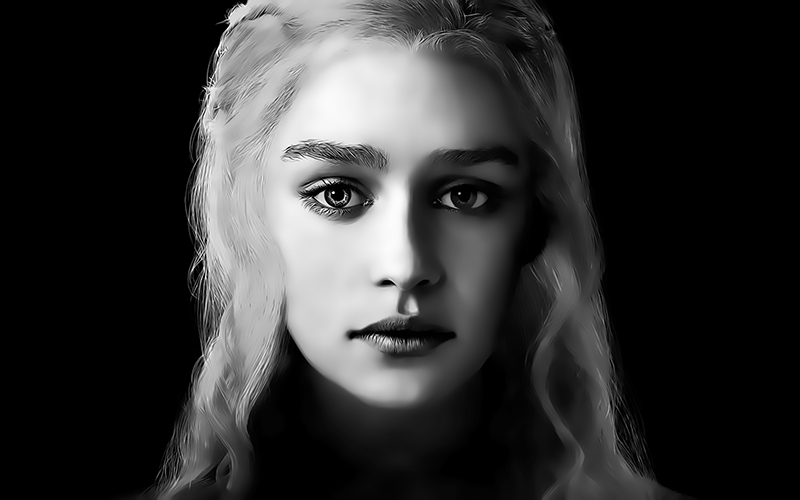This is a black and white portrait of a girl from the TV show Game of Thrones. The image has a striking composition, with her face positioned centrally and slightly angled, creating a dramatic light and shadow effect. Her face is half-illuminated by the light, highlighting her thick, dark eyebrows, one of which appears more pronounced due to the lighting. Her eyes, possibly brown, are accentuated with mascara and eye shadow, showing different shades due to the light's position. Her lips are full and prominent, with bright lipstick adding to the contrast in the monochromatic palette. She has wavy, blonde hair that's about shoulder length, which almost appears gray in the black and white setting. Her hair is parted in the middle, flowing gently to each side. The background is a deep, solid black, emphasizing the contours of her face and adding to the overall dramatic effect of the photograph. You can barely see her neck, which subtly emerges from the shadows, giving the portrait an ethereal and intense quality.